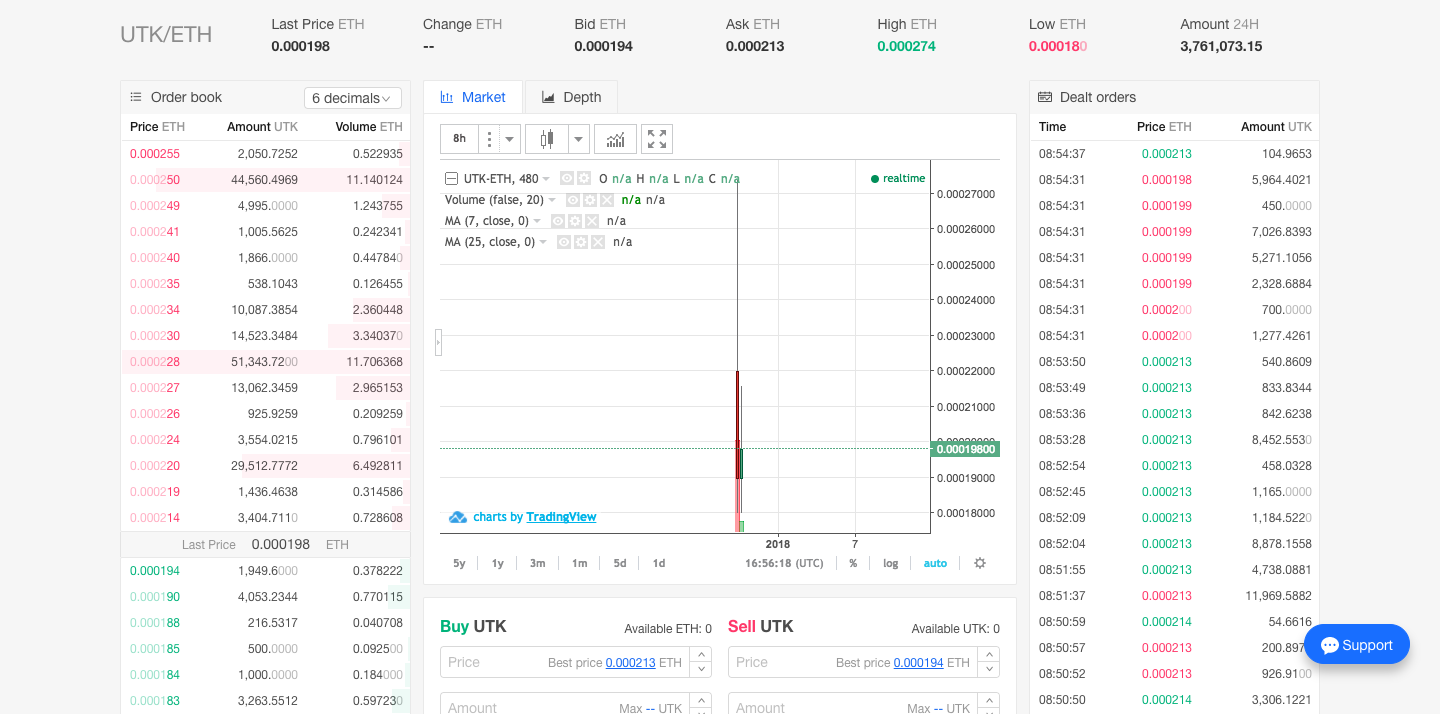This detailed caption would be:

"An intricate image showcasing a trading interface for cryptocurrency enthusiasts, particularly those interested in Ethereum (ETH) and UTRUST (UTK). The interface features a comprehensive chart displaying various statistics including the 'Last Price ETH,' 'Change ETH,' 'Bid ETH,' 'Ask ETH,' 'High ETH,' 'Low ETH,' and trading volumes within the last 24 hours. The data is visually organized using different colors, with pink, green, and other hues differentiating various numerical values. In the middle section, the screen displays live charts powered by TradingView, offering real-time price movements and trends. Additionally, a blue circular button labeled 'Support' in white text is positioned on the right-hand side, providing users with access to customer assistance for the trading platform."